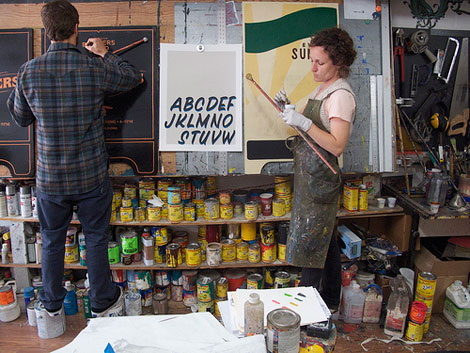In this color photo, two individuals are positioned in what appears to be a cluttered art studio. On the left side of the image stands a tall man with brown hair, dressed in a dark blue plaid shirt, denim jeans, and black and white sneakers. He is seen writing on a black chalkboard affixed to the wall, standing on two gallon paint cans, one under each foot. The chalkboard features an incomplete alphabet, missing some letters. Surrounding him are scattered paint cans and containers, creating a somewhat chaotic scene.

To the right of the image is a woman with curly brown hair, wearing a gray or brown rubber apron splattered with various colors of paint. Her short-sleeved shirt is peach in color. She is captured in profile, holding a large paintbrush and a container in one hand, with gloves on. Behind her and the man are three shelves filled with numerous jars and cans of paint, most with yellow labels, adding to the art studio ambiance. The floor is wooden, and the backdrop hints at a creative workspace, with the overall scene filled with vibrant shades of brown, gray, blue, green, orange, yellow, red, purple, light green, and light blue.